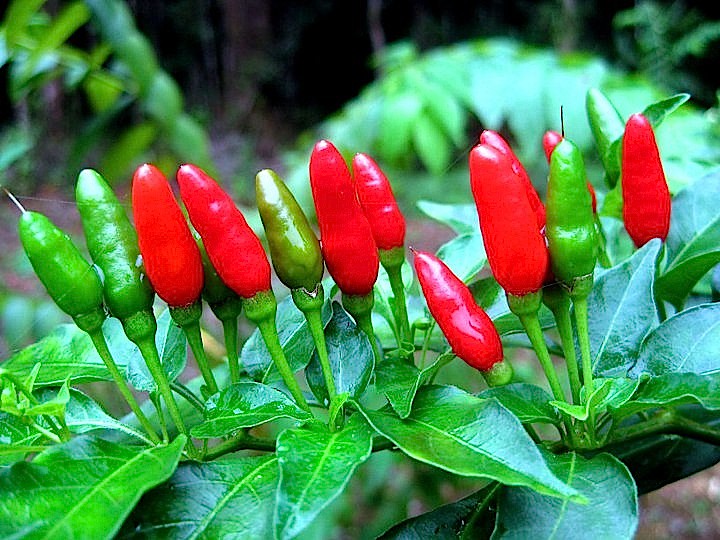This detailed color photograph captures a close-up of several peppers on their original plants, likely of a Chinese or Thai variety. The vibrant peppers, in shades of bright red and green, are pointed upwards with a slight tilt, and are arranged in a somewhat linear stack. Each pepper, elliptical in shape, is attached by green stems to a lush base of waxy green leaves adorned with light green veins. The composition includes pairs and trios of peppers, with two green ones followed by two red ones, then alternating green and red, creating a vivid and dynamic pattern. The background features an abundance of lush plant life, transitioning into a darker area that suggests the presence of trees or a dense, jungle-like canopy.